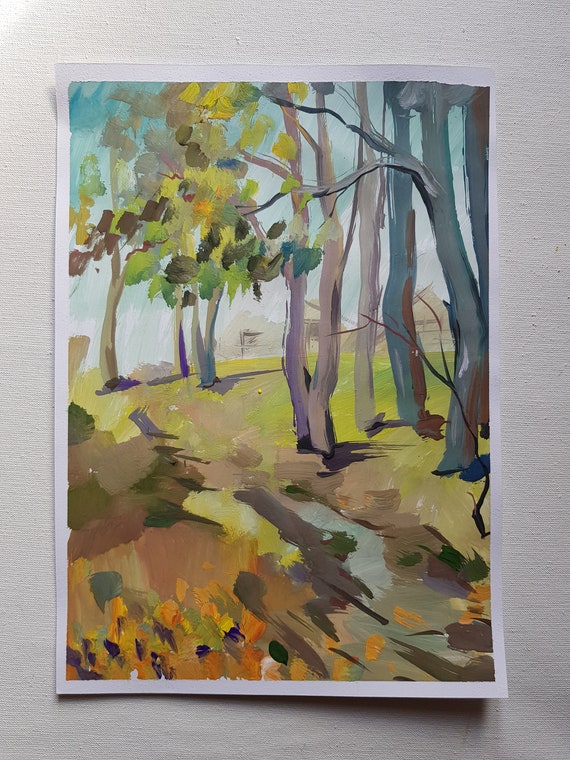This detailed, hand-crafted painting, likely created with pastel or watercolor and possibly finger-painted, is situated on a piece of special artistic paper, which in turn is mounted on a textured surface that resembles an artistic canvas. The painting depicts a slightly abstract outdoor autumn scene, characterized by its impressionist style with finger-width strokes. The scene features slender trees with thumbprint leaves, combining various vibrant shades of reds, yellows, greens, browns, and oranges to create a rich, seasonal palette. The ground is an amalgamation of these autumn colors, melding together with the suggestion of a pond or stream in muted blues and grays, which flows towards the right corner. In the background, there is a faintly visible homestead, adding a subtle layer of detail to the composition. The artwork exudes a simplistic charm, capturing the essence of a forest landscape in the fall, with bare and leafy trees standing tall against a blue sky.